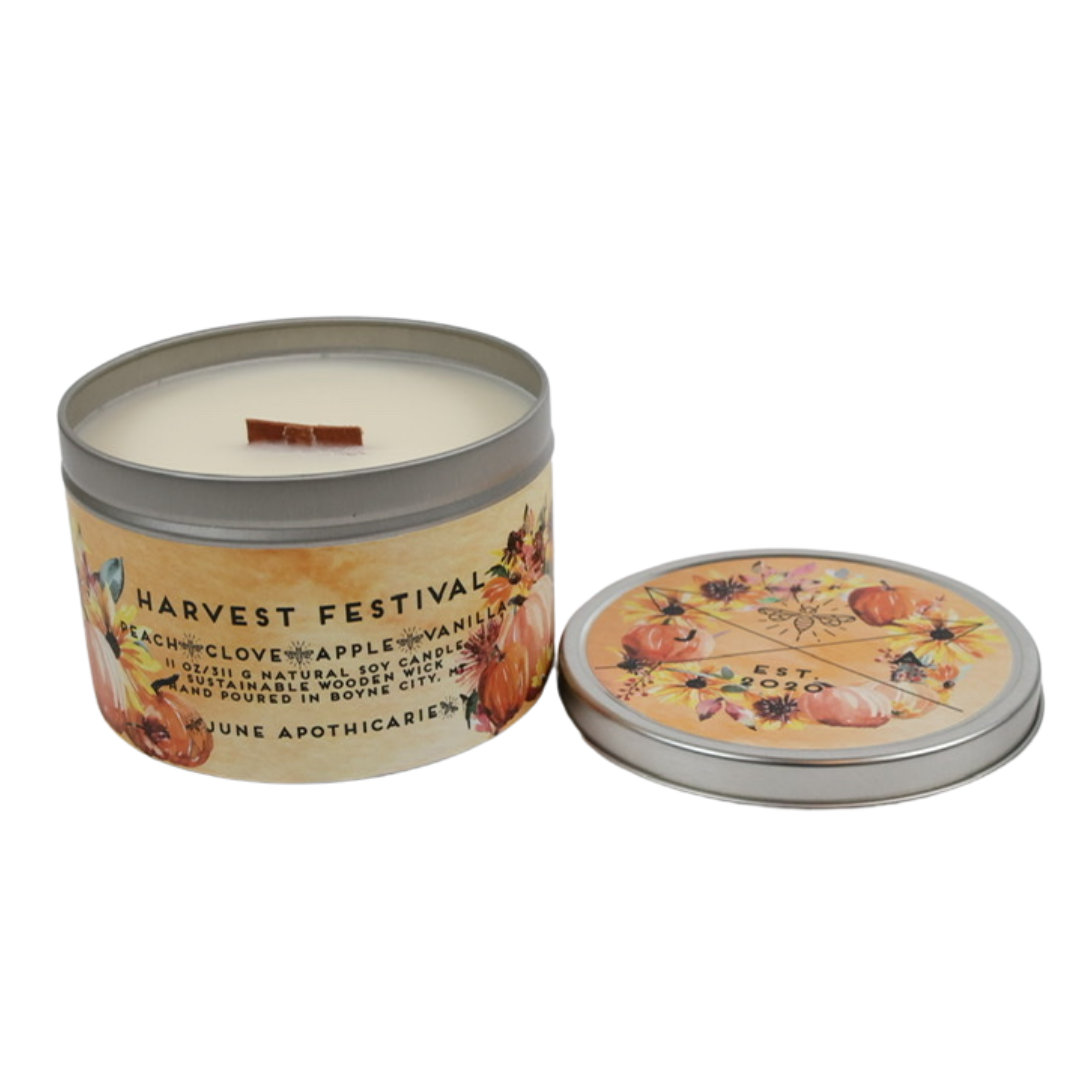This is a detailed photograph of a cylindrical, metal tin candle with its lid off, positioned to the right of the candle on a solid white background. The candle wax is white and features a dark orange wick. The tin has a decorative label with a sunburst background in shades of orange, adorned with illustrations of pumpkins, flowers, fruits, sunflowers, and a small bee. On the front of the tin, there is black text that reads "Harvest Festival," followed by "peach, clove, apple, vanilla." Additional text beneath includes "11 ounce, 311 grams, natural soy candles, sustainable wooden wick, hand poured in Boyne City, New Jersey," and "June Apothecary." The lid, which also lies near the candle, bears the text "est. 2020." The composition is clearly centered, with the candle facing forward, providing an inviting glimpse of its artisanal craftsmanship and autumnal theme.